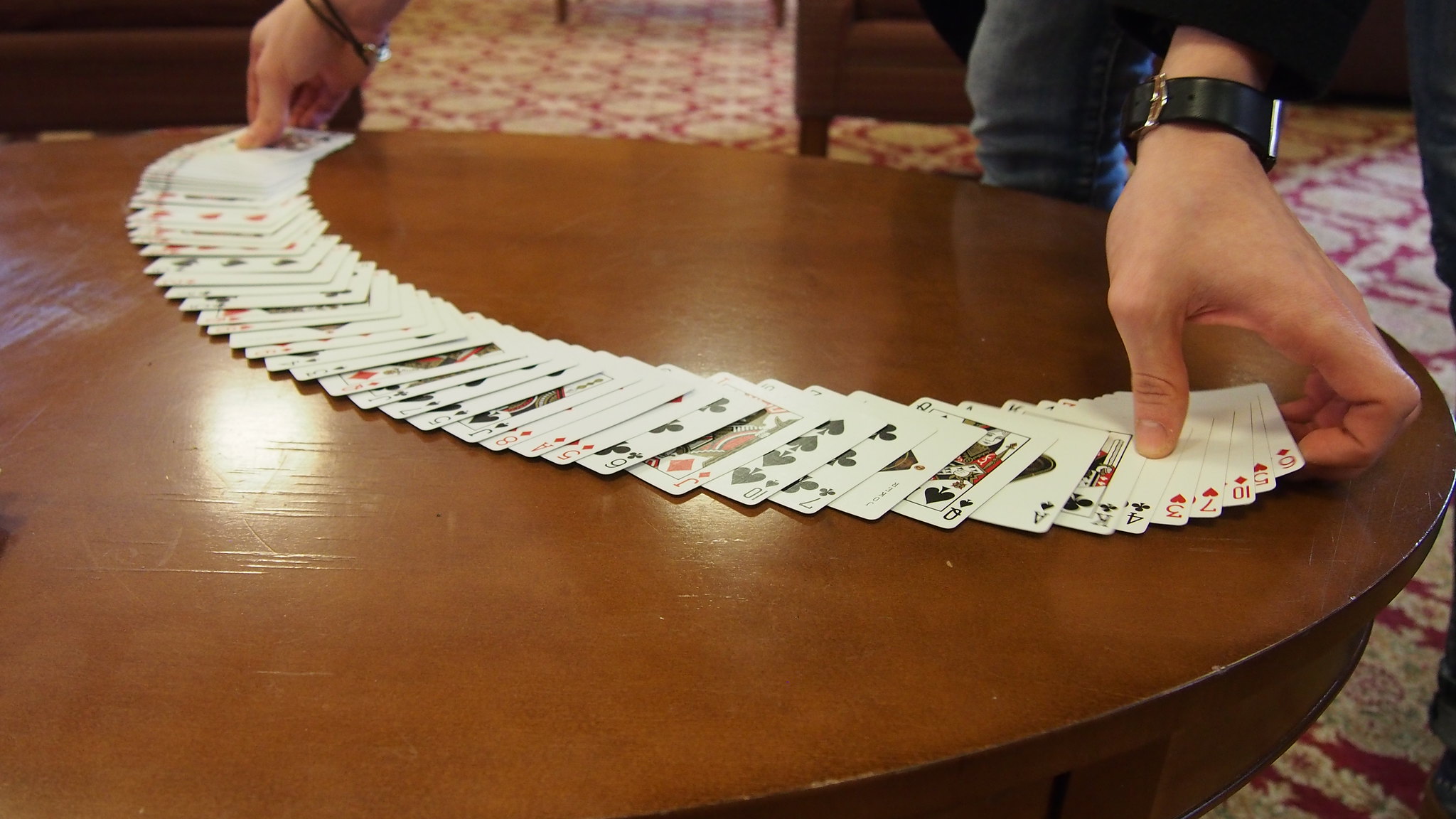In this image, the focus is on a meticulously arranged deck of cards being placed face-up in a semicircular pattern atop a circular wooden table. The subject's hands, likely belonging to a Caucasian male, are central to the scene. The left hand wears a watch with a black strap and silver details, while the right hand sports a thin black bracelet. Only the subject's legs, clad in denim trousers, are visible in the upper right corner of the frame. The background features chairs and a floor adorned with a white and red patterned motif, suggesting the setting could be a hotel or casino. The perspective of the shot offers an opposite viewpoint of the subject, emphasizing the care and precision in the card arrangement process.